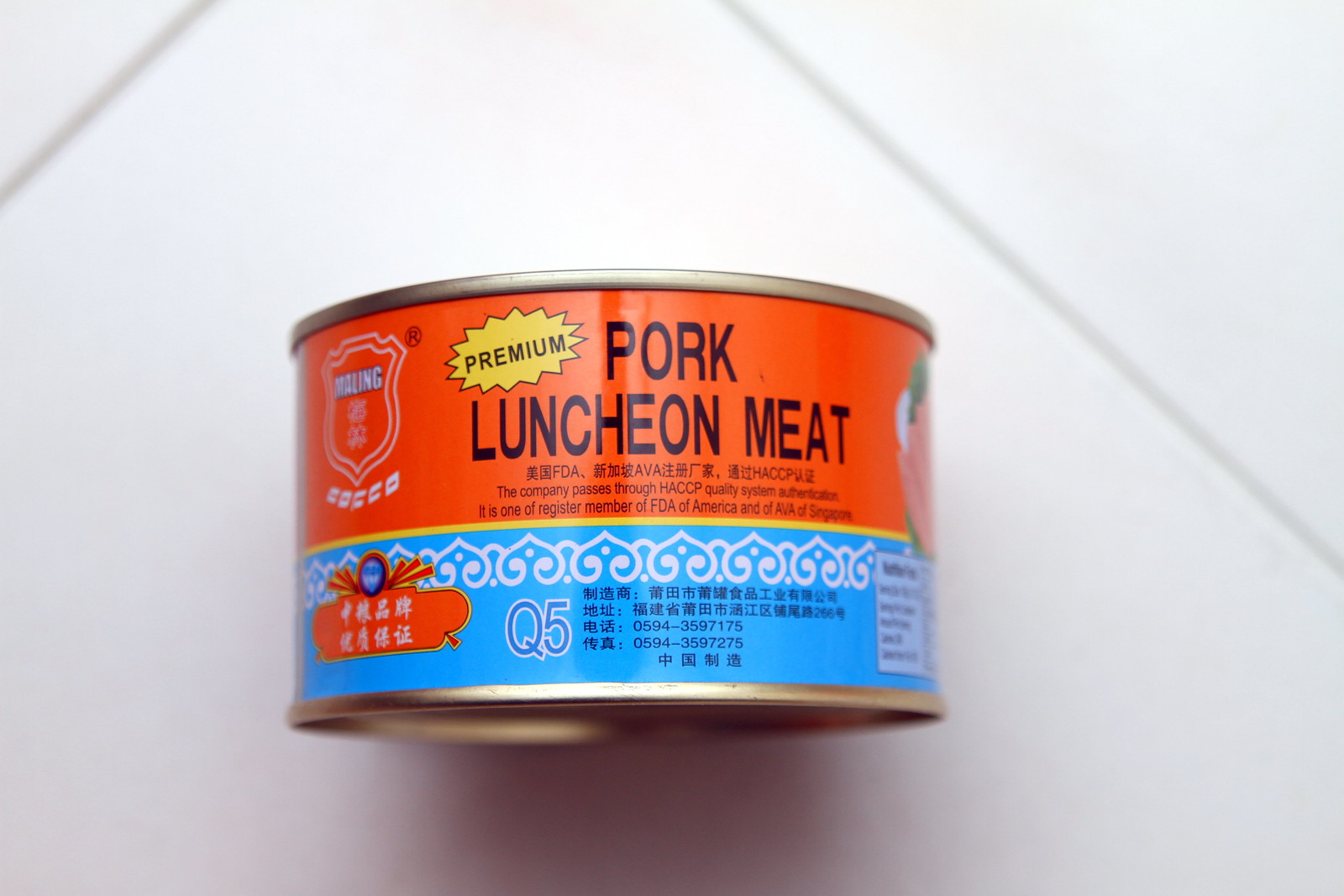This color photograph depicts a can of meat placed on a pristine white surface. The can prominently features a red label at the top with the text "Premium Pork Luncheon Meat." The top label also includes certifications, noting that the company adheres to the HACCP Quality System Authentication and is a registered member of the FDA of America and AVA of Singapore. Beneath the red label, a blue section adorns the can, showcasing a white geometric design and the text "Q5." The remainder of the text on the blue label is written in an unidentified Asian language. The image has a slightly wider-than-tall aspect ratio, with no people, animals, or buildings visible in the frame.